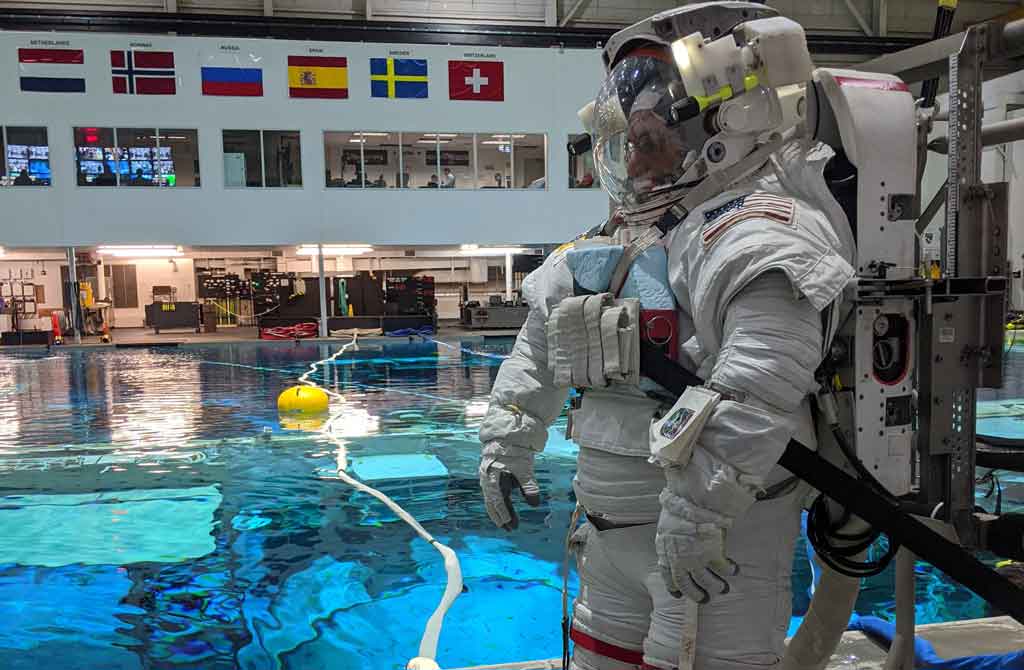In the photograph, a man wearing a bulky, white NASA space suit stands on a mechanical lift, poised to be submerged into a large, clear pool used for weightlessness training. His space suit is equipped with various attachments, including a large oxygen tank on his back, a transparent visor helmet, and a notepad positioned on his left arm. An American flag is visible on the left shoulder of his suit. Strapped to the front of his suit is a sponge, possibly for buoyancy. Surrounding the pool are numerous international flags, including those of Switzerland, Norway, and possibly the Netherlands and Scotland, among others. High above the pool, large windows provide a view into observation rooms where several people can be seen working. Throughout the pool, ropes and large yellow orb-like structures float, while submerged test structures can be seen beneath the surface, likely used for simulating various weightlessness scenarios. The facility is equipped with various pieces of equipment and storage areas, emphasizing its role in preparing astronauts for space missions.